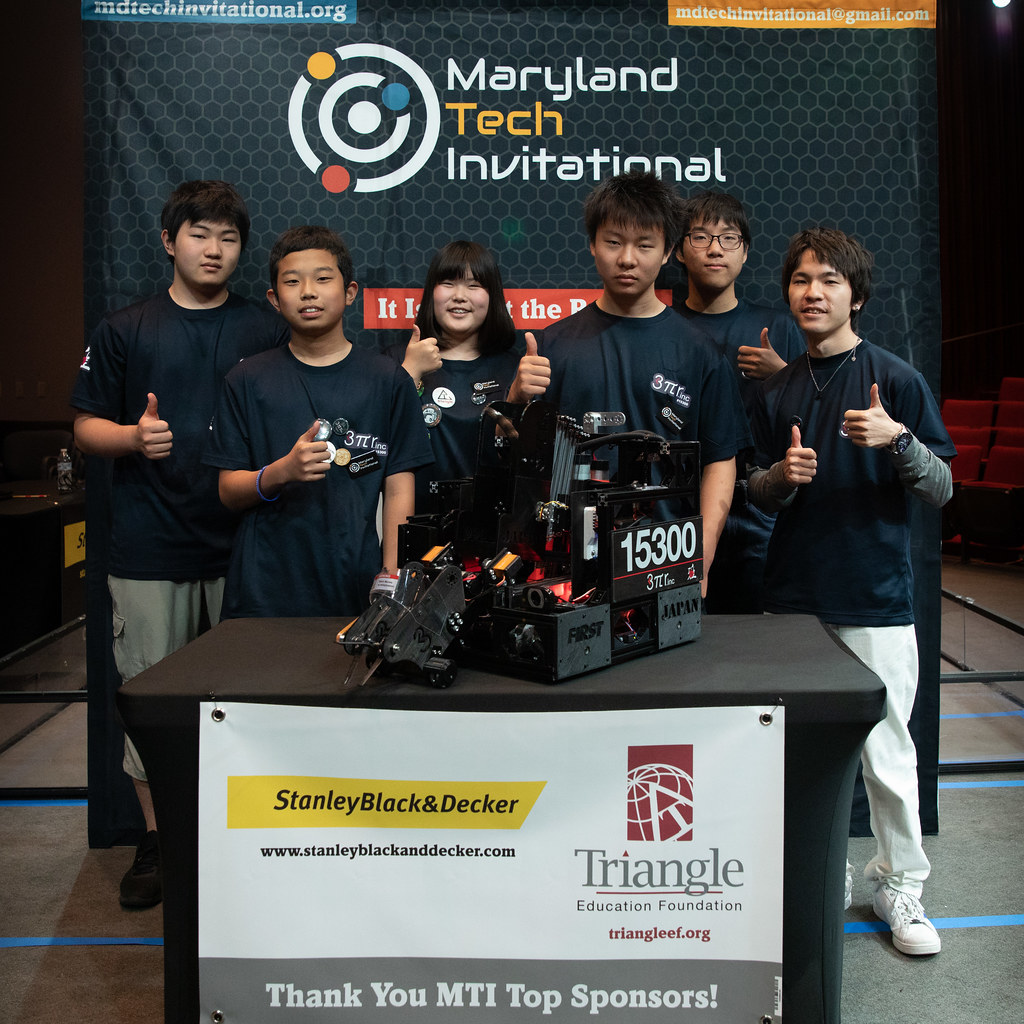This detailed photograph captures six Asian teenagers, five males and one female, standing in front of a sign that reads "Maryland Tech Invitational" with a gray honeycomb design. Each of them is dressed in matching black t-shirts and white pants, exuding team spirit. They are all giving thumbs up, with a mix of expressions ranging from smiles to serious looks. In front of them is a black table covered with a cloth, displaying a black robotic contraption identifiable by its arms, blades, and the numbers "15300" in white lettering. The contraption likely represents their entry in the competition. The table also prominently features a sponsorship banner that reads "Stanley Black and Decker, Triangle Education Foundation" with a website link "triangleaf.org" and the note "Thank You MTI Top Sponsors." This image encapsulates the essence of a tech-driven competition, highlighting the students' efforts and the supportive role of the sponsors.